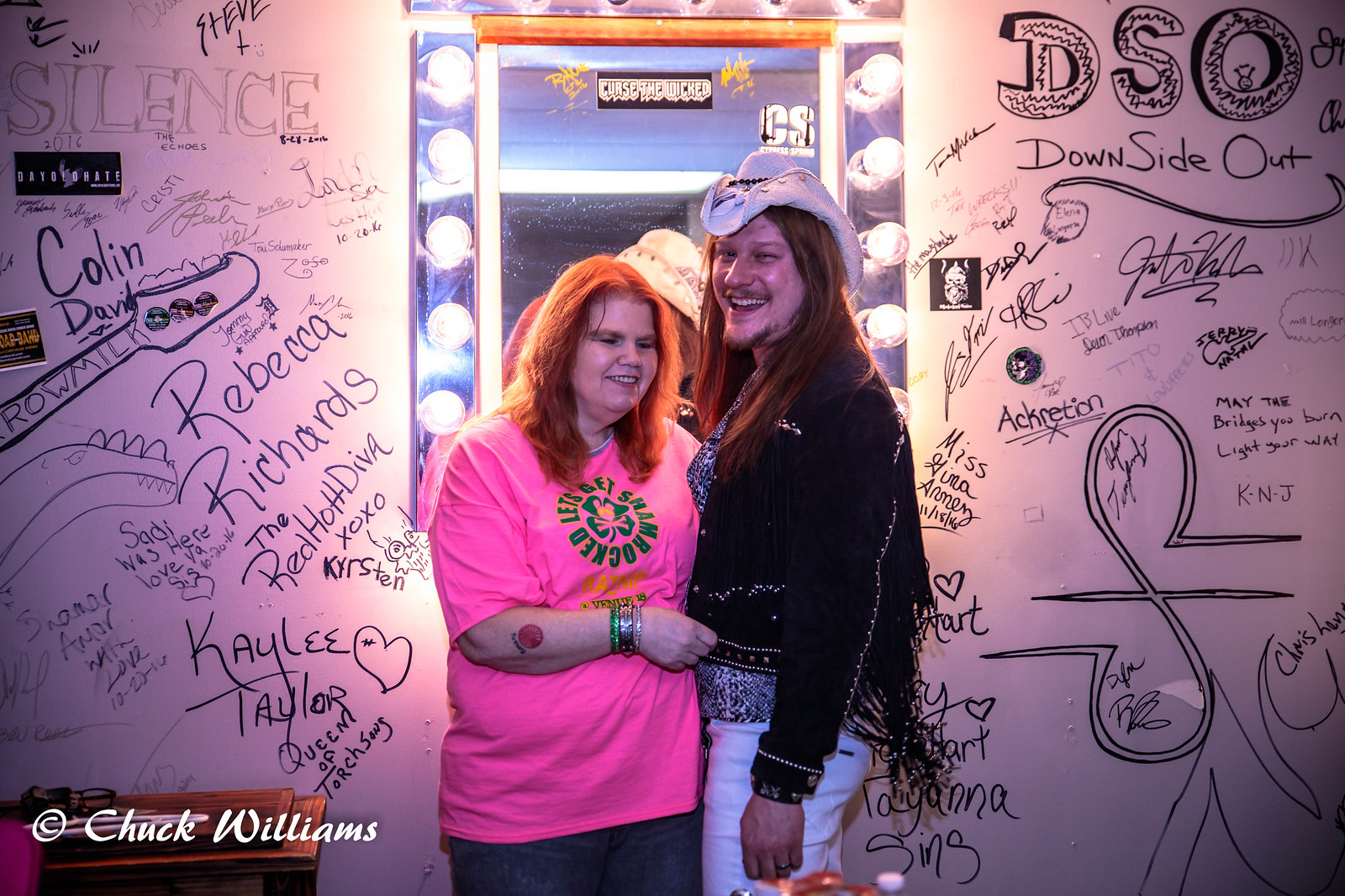This photograph captures two individuals standing in a room with distinctive decor. On the left, there's a woman with vibrant red hair cascading past her shoulders. She dons a pink t-shirt adorned with a green shamrock and blue jeans, with a red tattoo near her elbow. On her right, a man stands with long brown hair, a mustache, and a bit of a beard. He sports a distinctive curled-up cowboy hat, a black fringe jacket, a black and white shirt, and white pants. Both are smiling; she looks slightly to the side while he faces the camera.

Behind them, a silver-framed theater-style makeup mirror is prominently featured, its frame surrounded by glowing bulbs. The wall behind and around the mirror is cream-colored and densely covered with numerous signatures, diverse writings, and drawings, reflecting a vibrant tapestry of expressions. Notably, one of the larger inscriptions reads "DSO" with "Downside Out" in bold block letters. At the bottom left corner of the image, the photographer's name, Chuck Williams, is credited, adding an official touch to the lively scene.